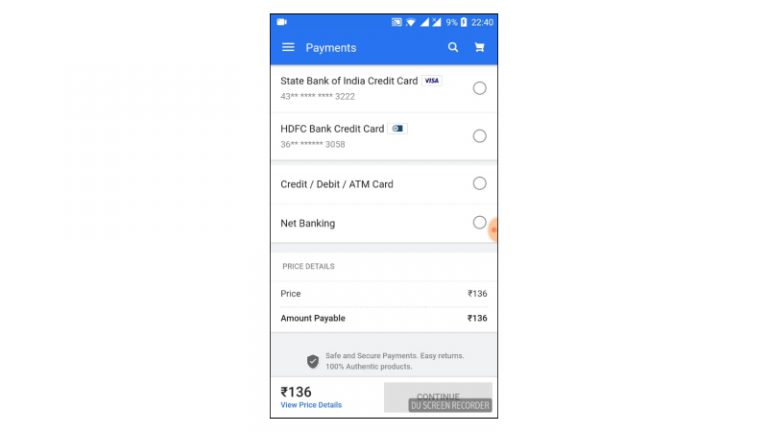The image, captured from a cell phone screen, displays a digital payment application. At the top of the screen, a solid blue bar contains various icons. On the right-hand side, the time is prominently displayed as "22:40." Adjacent to the time, a fully charged battery icon shows a white battery outline with a black lightning bolt inside, indicating that the phone is currently charging.

On the left side of the blue bar, there appears to be an icon resembling a video camera. Below this section, a white header with three horizontal white lines on the left and icons of a magnifying glass and a shopping cart on the right, indicates a navigation menu. The header text reads "Payments."

The main content of the screen lists details of two credit cards. The first entry is labeled "State Bank of India Credit Card" accompanied by a Visa logo. The card's partial number is displayed as "43** **** **3222," with asterisks obscuring the middle digits for security reasons.

The second entry indicates an "HDFC Bank Credit Card" with a smaller card icon next to the text. The card's partial number is shown as "36** **** **** 3058," similarly obscured with asterisks.

The screen continues to list similar information for other cards beneath, maintaining the same format and style.